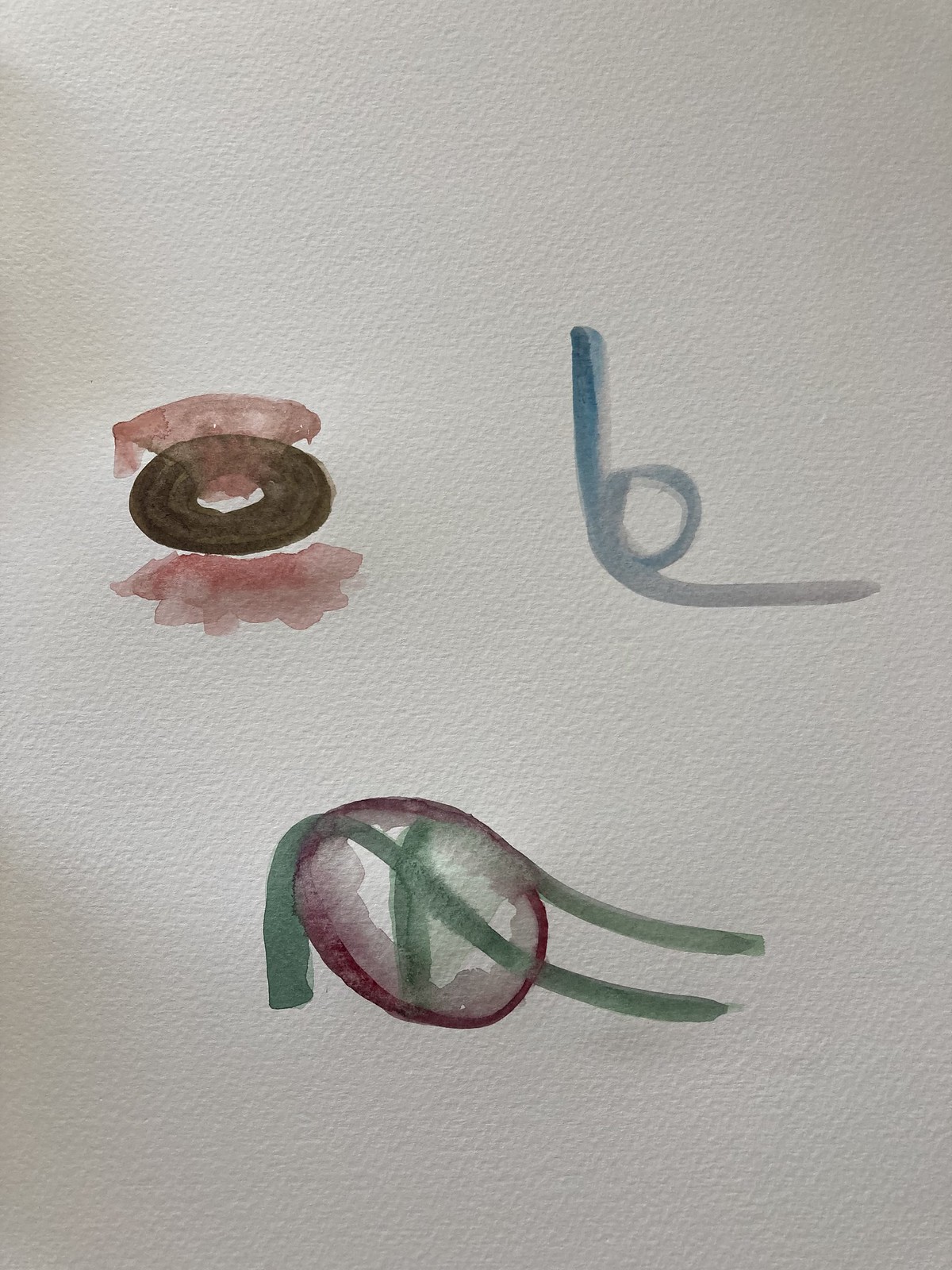This photograph captures a beautifully detailed watercolor painting on a piece of white, textured watercolor paper. The paper's toothy ridges are noticeably visible. The painting features three distinct shapes. In the upper left corner, there's a brown donut-like ring with a slightly darker hue adding to its texture, accompanied by transparent pink clouds above and below it. To the right, a blue and gray curvy line starts with a darker shade of blue, curving down to the left and forming a loop in the center before extending horizontally. At the bottom, there is a red and white circle resembling a large slice of onion, crisscrossed with green lines that add an intricate overlay to the shape. Each element combines to create an abstract, yet harmonious composition that’s both visually intriguing and richly textured.